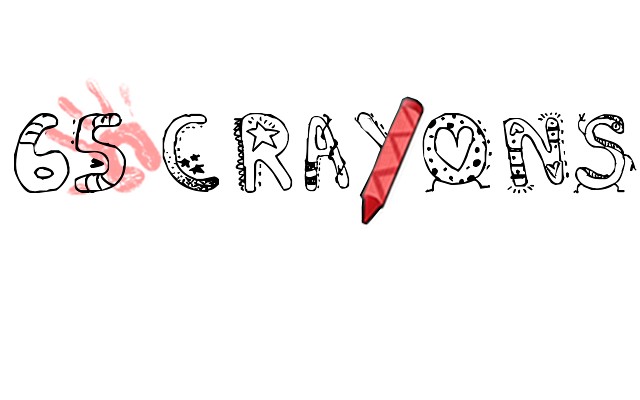In the image set against a plain white background, the text "65 crayons" spans the center. This text appears hand-drawn, with each character uniquely embellished. The number "65" is marked with three lines on top of both digits, while the digit "5" overlays a red handprint, resembling a child’s hand pressed with paint. The "C" in "crayons" is adorned with three stars and polka dots, the "R" features a star in its loop, and the "A" has stripes on one leg and what looks like a cord spiraling around the other. The "Y" is creatively formed from a red crayon, the "O" houses a heart in its center with two small legs at the bottom, the "N" is decorated with stripes and hearts, and the "S" has two legs and two waving arms. The entire composition gives off a playful, child-like vibe, reminiscent of a whimsical drawing or a potential logo for a kid-focused brand.